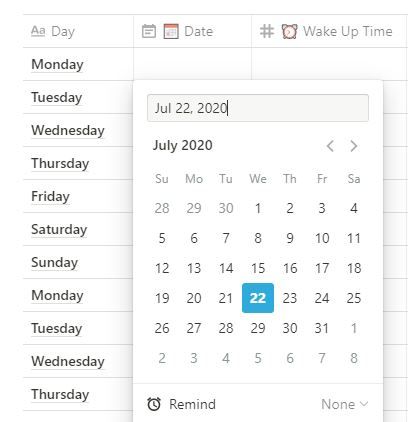The image features a detailed, digital calendar interface set against the backdrop of a spreadsheet-like layout. At the top of the calendar, inside a rectangular box, the date "July 22, 2020" is prominently displayed. Just below this box, the text "July 2020" appears in bold black. To the left and right of this text are navigational arrows, enabling the user to move between months.

The calendar grid underneath features the days of the week—Sunday through Saturday—in a horizontal row, with each corresponding date for the month of July 2020 listed beneath each day.

At the bottom of the calendar section, there is an alarm icon symbolizing reminders. Adjacent to it, the text "None" is displayed, indicating that no alarms are currently set. To its right, there is a downward arrow, hinting at the possibility of expanding or diving into a subcategory.

Below the calendar, the layout transitions into a spreadsheet-like format. This section includes columns labeled "Day," "Date," "Number," and "Wake Up Time" with another alarm icon next to "Wake Up Time." The "Day" column includes an underlined capital "A" followed by an underlined lowercase "a," suggesting some alphabetical ordering or importance.

Each day, from Monday through Sunday, is listed sequentially with the initial letter capitalized. The sequence repeats, indicating that it may cover more than a single week. The text format, layout, and visual cues all work together to resemble a systematic approach to scheduling and data management.